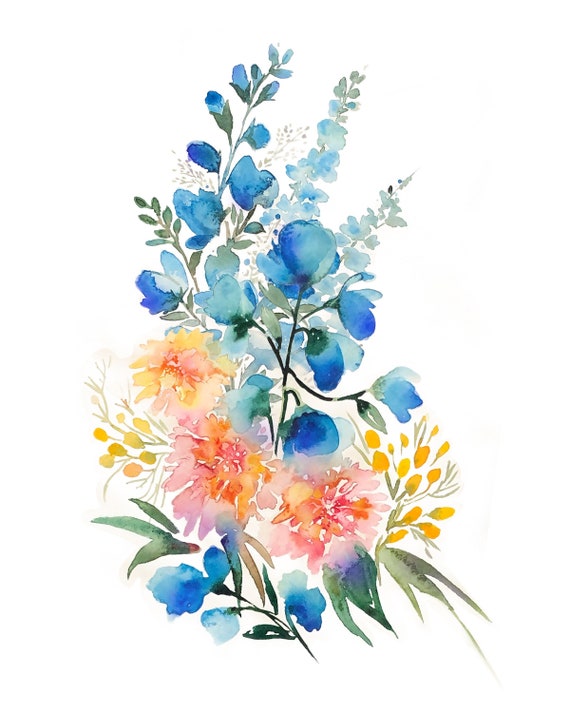The artwork is a detailed watercolor painting on a stark white background, depicting a vibrant bouquet of flowers. At the top of the image, there are four tall, narrow stalks bearing blue flowers that closely resemble blue bonnets. The central stalk is in the foreground, showcasing a vivid blue hue, while the other three stems feature more muted blue tones and are partially in the background. Green stems are interwoven with these blue blooms, some of which also display buds yet to open.

Beneath these blue stalks, the middle portion of the painting transitions into warm hues of pink, orange, and yellow. This area features three wide, circular flowers that exude the vibrant colors of a sunset. Surrounding these are smaller, yellow filler flowers that have a sage-like appearance. Dark green leaves frame the bouquet in the lower corners.

The bottom section of the painting contains another set of blue bonnets, providing a cohesive balance to the composition. The interplay of vibrant and muted colors, along with the delicate details of the flower petals, stems, and leaves, creates a harmonious and captivating piece.